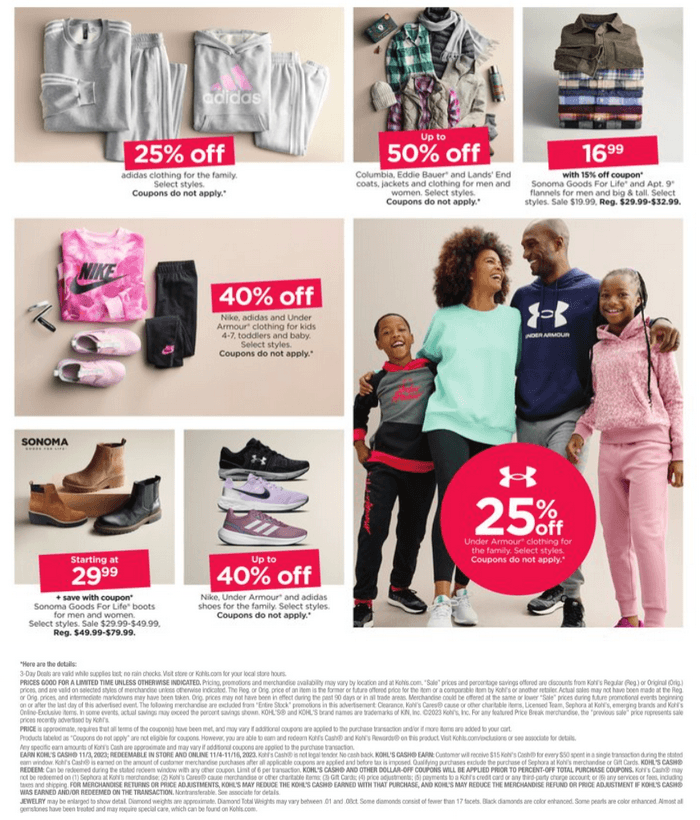Get ready for incredible savings on family clothing with deals up to 50% off! Highlighted items include a stylish gray sweater, now available for up to 50% off, and a pink shirt from Nike. You'll find great deals on renowned brands such as Columbia, Eddie Bauer, Nike, Adidas, and Under Armour, with special discounts like 40% off on kids' clothing. Families can also enjoy $16.99 offerings and Sonoma goods priced between $6.99 and $29.99. Featured selections include jackets and clothing for men and women, plus options for children. Look out for the black, red, and blue shirts, dark sweaters, and footwear like brown and black shoes. Don't miss the displayed coupons to maximize your savings at checkout!